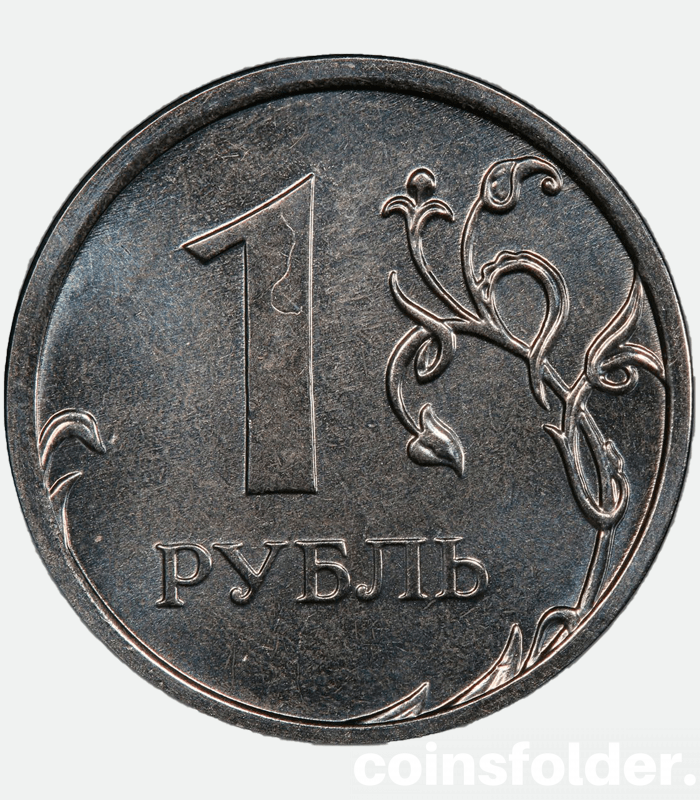In this image, a singular coin dominates the central focus, set against a plain gray background. The coin is silver in color and appears to be of foreign origin, possibly part of someone's personal collection. Accompanying the image is a watermark in the bottom right corner that reads "coins folder," with no additional text visible. The coin itself features the number "1" prominently displayed, which has a distinctive vertical scratch resembling a fish hook in its upper half. Below the number, the letters "P-Y-E-J-I-B" are inscribed. To the right side of the coin, a detailed vine design twists and branches out into three different ends. The coin is round and encircled by a slightly protruding lip, or ridge, around its edge. Though it shows some signs of wear, such as the scratch on the number and a minor crack, it remains in relatively good condition considering its apparent age. The overall color palette of the coin includes shades of gray, white, dark gray, and black.